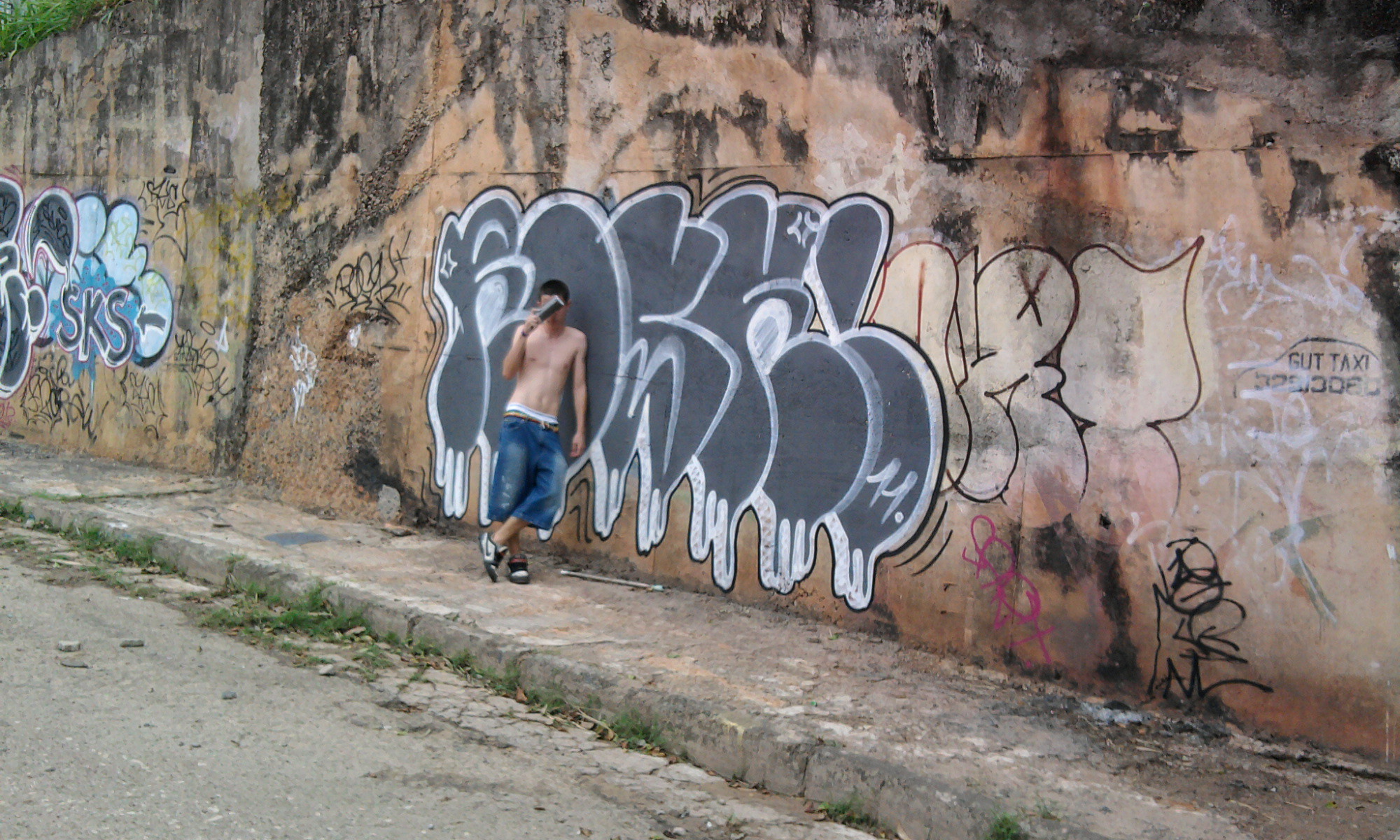In this photo, a young, thin boy with short hair leans casually against a graffiti-tagged wall, his face obscured by a rolled-up magazine. He stands with one leg crossed over the other, showcasing his relaxed posture. The boy is bare-chested, revealing his white and grey boxers peeking out from beneath very low-rise, wide-legged jean shorts that reach mid-calf. A belt loosely cinches his shorts, and he wears black and white running shoes without socks.

The graffiti wall behind him transitions from a light brown shade at the bottom to a darker grey at the top and features various tags and texts. Prominent among the graffiti are black letters with white at their base, exuding a dripping effect as though the paint were still wet. Further up the street, another piece of graffiti displays light grey and white clouds along with the letters "SKS" in grey. The broken cement walkway in front of the wall is old and cracked, and leads up to the dark, cracked paved road, creating an urban, somewhat decrepit scene. Overall, the image captures a gritty slice of city life, highlighting the juxtaposition of youthful nonchalance and urban decay.